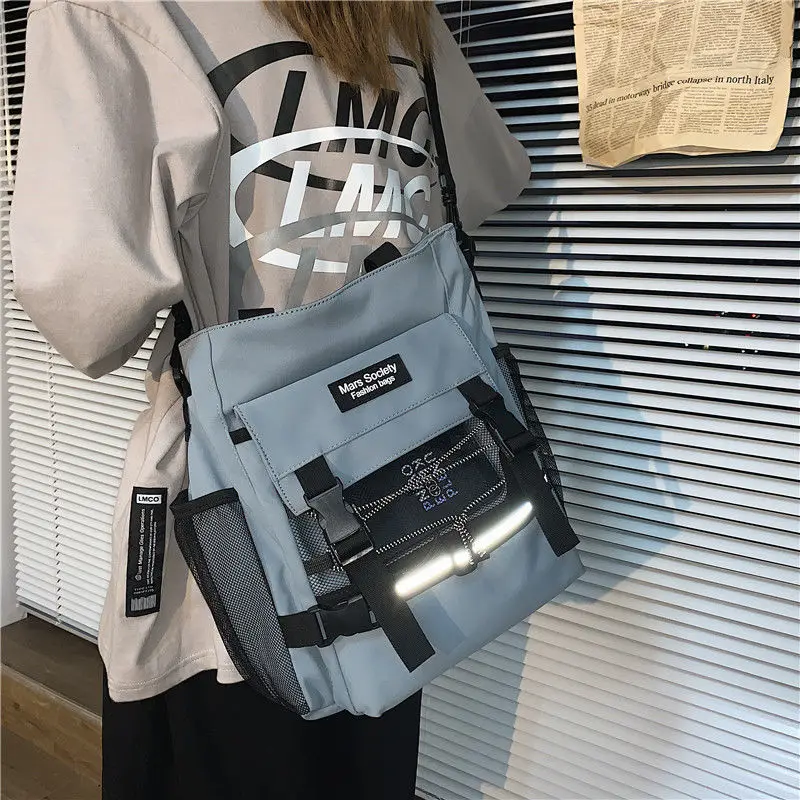In this image, a woman is modeling a stylish light blue backpack with black straps and buckles, positioned over her lower back. She is captured from the knees up, with her head cropped out of the frame. She wears an oversized grey t-shirt with the text "LMC" on it and a pair of black pants. Her brown hair is partially visible. The backpack, which resembles a messenger bag, has a front flap with clasps, a mesh side pocket for water bottles, and bears a label that reads "Mars Society Fashion Bags." There is also a light strip on the bag, adding an interesting detail. The background features white blinds with an old newspaper attached to them on the upper right and a wooden platform below, grounding the scene. Her pose and the setting create a casual, yet stylish presentation of the bag.